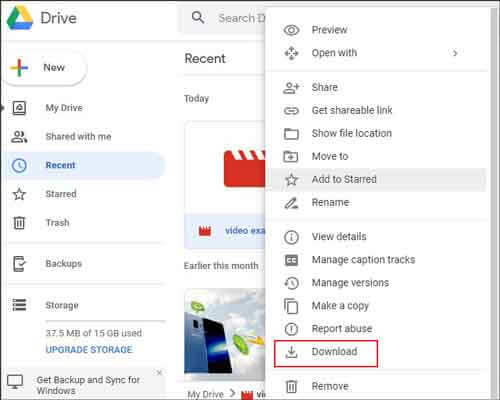This image showcases a Google Drive interface. On the far left, a vertical sidebar features the primary "Drive" tab, directly right of which is a gray portion of the search bar. Below "Drive," the sidebar displays several labels: "New" with a multi-colored plus sign in green, red, yellow, and blue, followed by "My Drive," "Shared with Me," and the currently selected "Recent" tab highlighted in blue. Following this are tabs for "Starred," "Trash," "Backups," and "Storage," indicating "37.5 MB of 15 GB used" with an option to "Upgrade Storage." Below this segment is a link to "Get Backup and Sync for Windows."

To the right side of the sidebar, the main content area shows the "Recent" section, starting with a subheading "Today." Below this subheading is a cropped view of what appears to be a video file, followed by an image depicting an open door with a sky background.

On the far right, a vertical pop-up with a white background lists numerous options from top to bottom. These options include "Preview," "Open With," "Share," "Get Shareable Link," "Show File Location," and "Move To." "Add to Starred" is highlighted. Additional options shown are "Rename," "View Details," "Manage Caption Tracks," "Manage Versions," "Make a Copy," "Report Abuse," and "Download," the latter of which is distinctly marked with a red rectangular border. The final option in the list is "Remove."